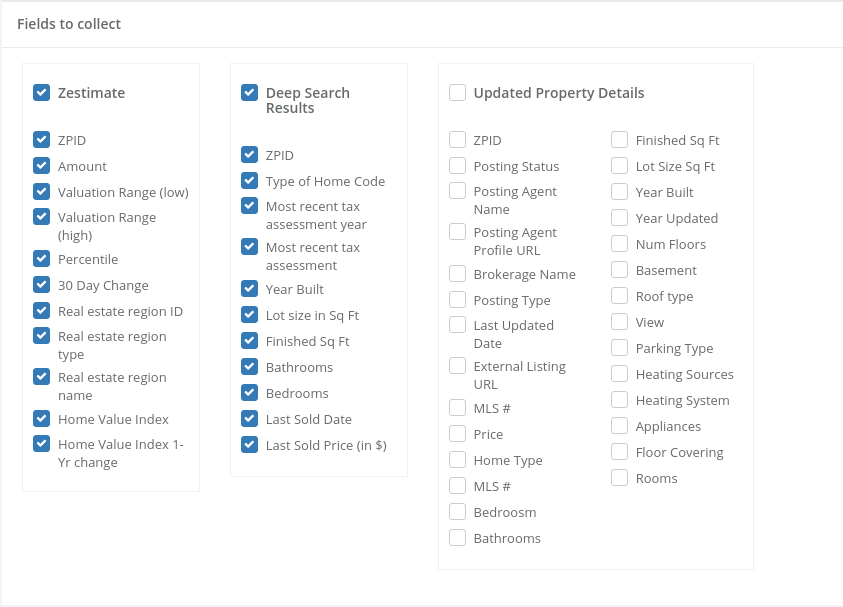**Image Description: Detailed Data Selection Interface**

The image is a landscape-oriented rectangle typical of web page layouts, predominantly featuring four columns of selectable checkboxes aligned with text entries. The background is completely white, with all text rendered in varying shades of medium to dark gray. A thin gray border outlines the top, left, and bottom sides of the image, leaving the right side borderless.

At the top left corner, there is a bold header reading "Fields to collect," with only the "F" capitalized. This header occupies about 10% of the image's height and is underlined to separate it visually from the rest of the content below.

Beneath this header, the main content area contains three portrait-oriented rectangles distributed across four columns, with the rightmost rectangle spanning two columns. These rectangles are bordered by very thin gray lines and contain lists of checkable items, all left-justified.

**Left Column:**
- **Header:** Bolded text "Zestimate" followed by a blue checkbox with a white checkmark.
- **Entries (All checked):**
  1. ZPID
  2. Amount
  3. Valuation Range (Low)
  4. Valuation Range (High) (wraps to a second line)
  5. Percentile
  6. 30 day change
  7. Real Estate Region ID
  8. Real Estate Region Type (wraps to a second line)
  9. Real Estate Region Name (wraps to a second line)
  10. Home Value Index
  11. Home Value Index 1-Year Change (wraps to a second line)

**Middle Column:**
- **Header:** Bolded text "Deep Search Results" with "Results" on a second line.
- **Entries (All checked):**
  1. ZPID (all caps)
  2. Type of Home Code
  3. Most Recent Tax Assessment Year (wraps to a second line)
  4. Most Recent Tax Assessment (wraps to a second line)
  5. Year Built
  6. Lot Size in SQFT
  7. Finished SQFT (abbreviated without periods)
  8. Bathrooms
  9. Bedrooms
  10. Last Sold Date
  11. Last Sold Price (in dollar sign)

**Rightmost Columns (Spanning Two Columns):**
- **Header:** Bolded text "Updated Property Details"
- **Entries (none checked, arranged in two columns):**
  - **Left Column:**
    1. ZPID
    2. Posting Status
    3. Posting Agent Name (wraps to a third line)
    4. Posting Date
    5. Listing Price
    6. Property Type
    7. Property Use
    8. Year Built
    9. Lot Size
    10. Living Area
    11. Bathrooms
    12. Bedrooms (misspelled as "Bedroosm")
    13. MLS# (pound sign indicates the field is for numbers)

  - **Right Column:**
    1. Finished Square Feet (abbreviated as SQFT)
    2. Rooms

The design emphasizes easy interaction through clickable checkboxes with a clean, minimalist aesthetic. Each section is well-organized, with clearly defined headers and logical groupings of related data fields.